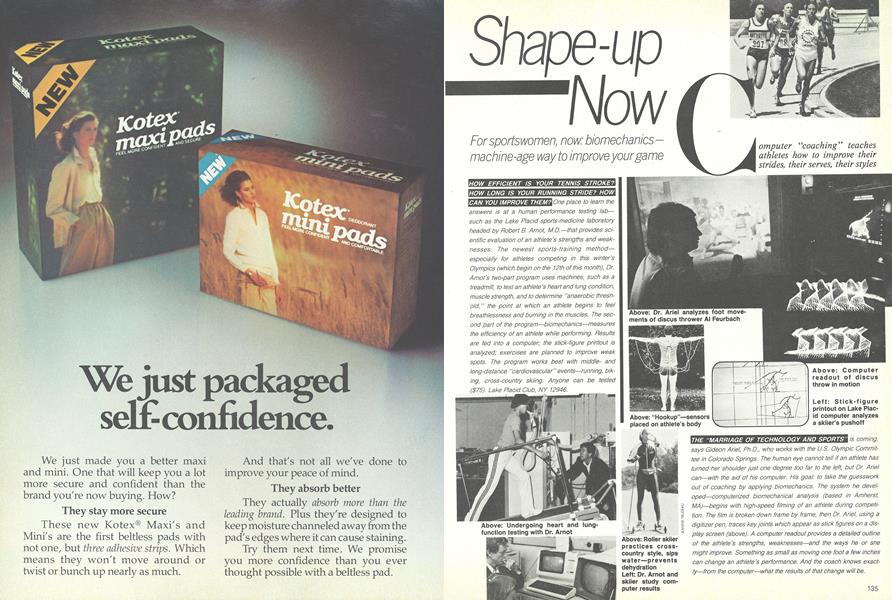The image depicts a two-page magazine spread. The left page features an advertisement for Kotex pads, prominently showcasing two product boxes, one for MaxiPads and the other for MiniPads. Each box has a banner in the upper left corner indicating the product is "new." The left box, adorned with imagery of green trees, features a woman with her hands in her pockets, dressed in a collared shirt. The right box, set against a backdrop of tall brown grass, shows a woman in a white shirt and light-colored pants. The caption beneath reads, "We just packaged self-confidence," followed by descriptive paragraphs about the products.

The right page presents an article titled "Shape Up Now," geared towards sportswomen. This black and white page discusses biometric ways to improve physical fitness and performance. It includes several images of women engaged in physical activities—one using a treadmill and another analyzing information on a computer screen—with detailed paragraphs explaining the content and benefits of biometrics in sports training. The article begins with a large initial "C."